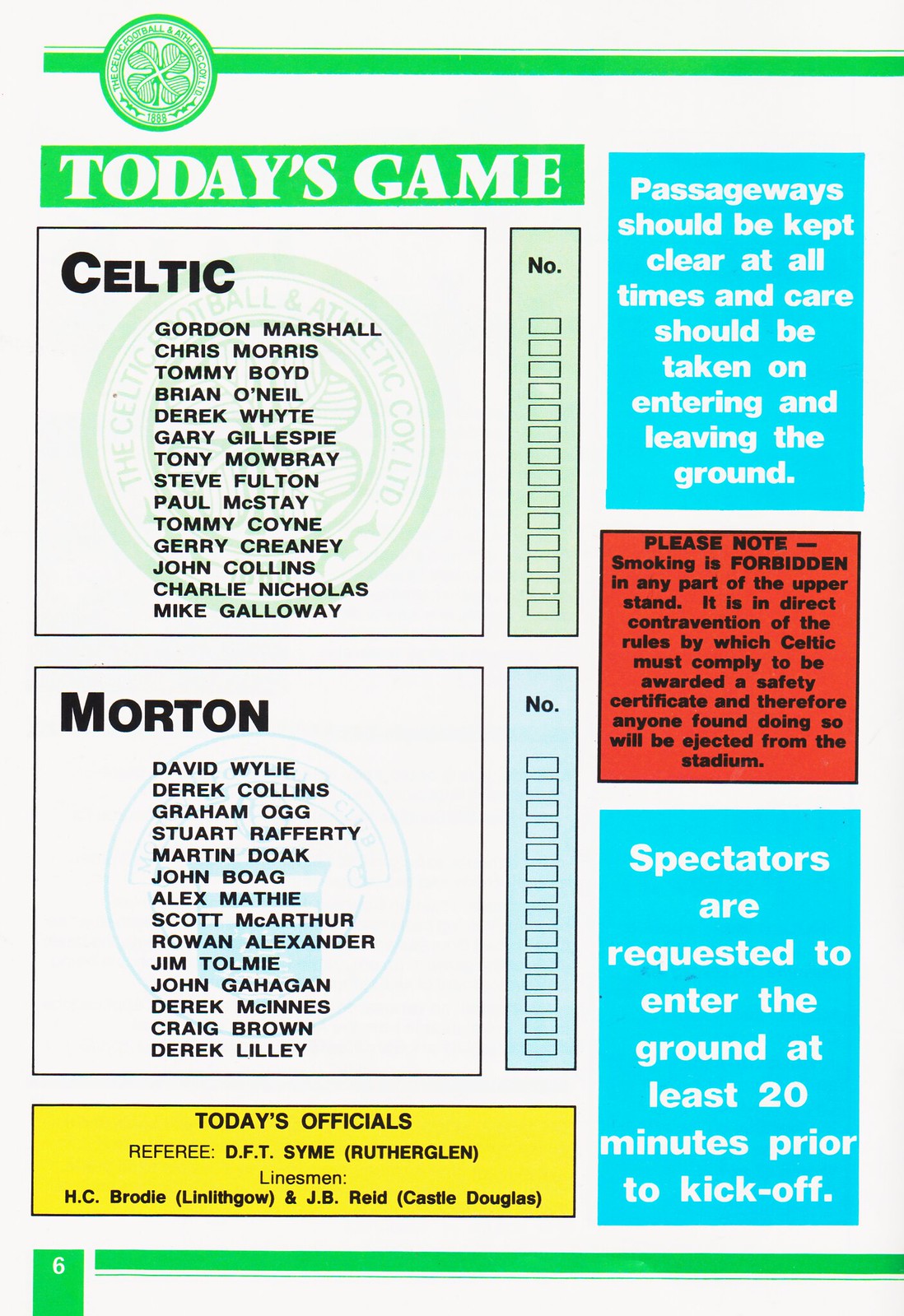This colorful poster, akin to a magazine graphic, details the players and ground rules for a soccer match between Celtic and Morton. At the top of the poster, there's a green rectangle featuring an insignia on the left corner and white text that reads "Today's Game." Below, the teams' names, Celtic and Morton, are highlighted in black against a white background, each followed by a vertical list of players for both teams.

For the Celtic team, players listed include Gordon Marshall, Chris Morris, Tommy Boyd, Brian O'Neill, Derek White, Gary Gillespie, Tony Mowbray, Steve Fulton, Paul McStay, Tony Coyne, Jerry Cranie, John Collins, Charlie Nicholas, and Mike Galloway.

To the right, three blue rectangles provide key information and rules for spectators, such as "Spectators are requested to enter the ground at least 20 minutes prior to kickoff," "Passageways should be kept clear at all times," and "Care should be taken on entering and leaving the ground." Additionally, there is a red and black warning that smoking is forbidden. At the bottom of the poster, in yellow text, it lists today's officials, including the referee and linesmen.

In summation, this comprehensive poster outlines the players, officials, and essential guidelines for attendees at the match, ensuring a clear and organized event.